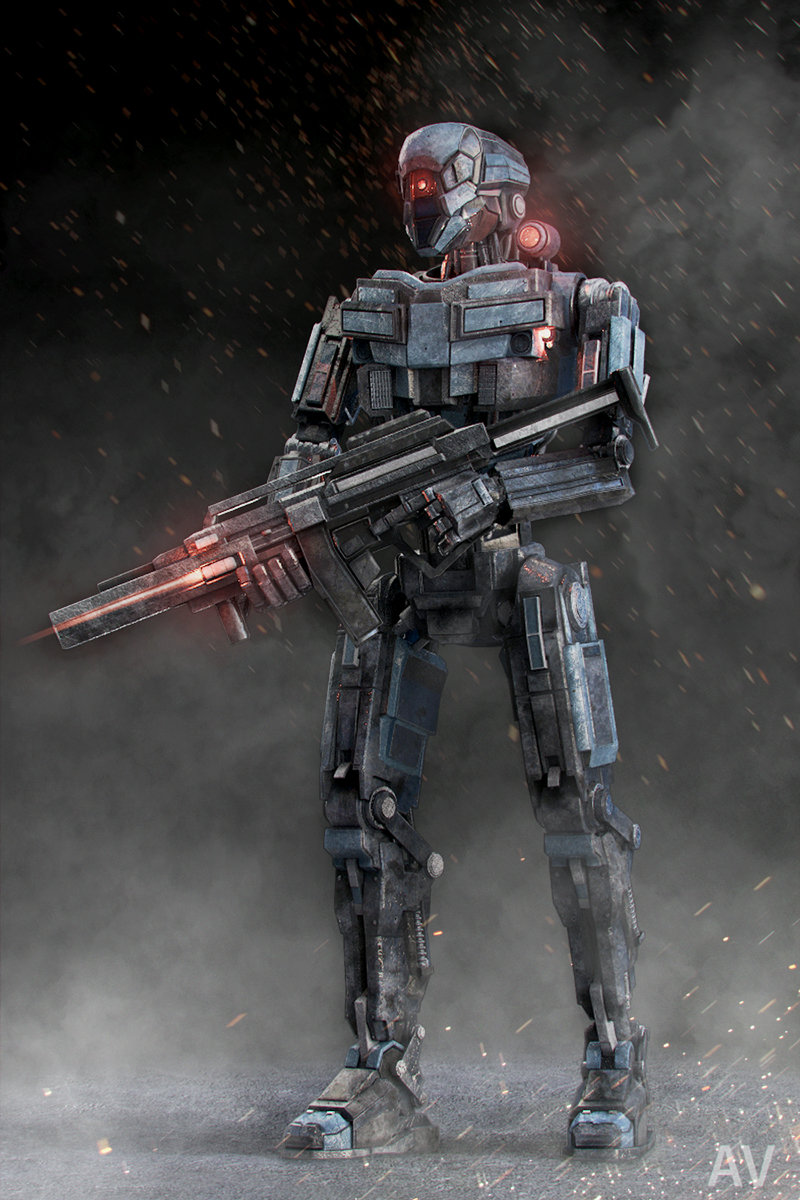The illustration portrays a highly detailed, futuristic military robot set against a gray and black smoky backdrop, punctuated by sparks and raindrops. The robot, clad in silver metal from head to toe, features a singular, ominous red eye in the center of its forehead and additional red light accents on its right shoulder and weapon. The robot is armed with a sleek, gray-black machine gun with red and black detailing, from which a red beam of light emanates. The robot stands in a dynamic pose, gripping the gun with both hands—its left hand near the trigger and its right hand supporting the barrel. In the lower corner of the image, the letters "A.D." or "A-V" are prominently displayed in white, adding a cryptic element to the scene.